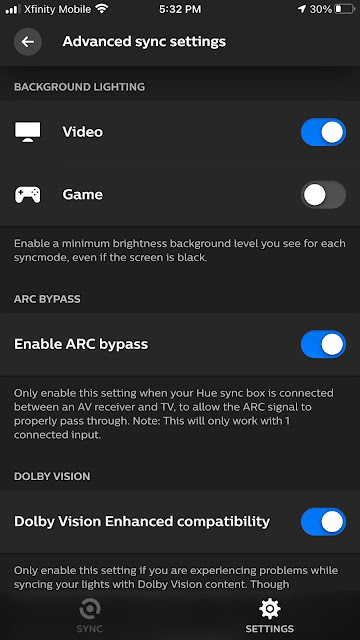**Detailed Caption:**

The screenshot displays a configuration menu on a device, likely a smartphone or tablet, with a black background and white text. At the top of the screen, the heading reads "Advanced Sync Settings." The screenshot reveals several configurable options:

1. **Video** - This option is checked.
2. **Game** - This option is left unchecked.
3. **Enable Minimum Brightness** - The reason for this setting leads us to believe that the content is tailored to a video device.

Further down, the screenshot shows the "ARC Bypass" setting enabled, with a note specifying: "Enable this setting when your Hue Sync Box is connected between the AV receiver and TV."

Additionally, "Adobe Vision" is enabled, with instructions stating: "Enhance compatibility. Enable this only if you are experiencing problems while syncing your lights with your Adobe Vision content."

At the very bottom of the settings menu, there is an indicator that the sync feature is not currently activated, as the sync button is not enabled. Overall, this screenshot encompasses various sync settings, highlighting options to sync video, enable ARC bypass, and enhance compatibility with Adobe Vision content, aimed at improving the lighting experience in tandem with video playback.